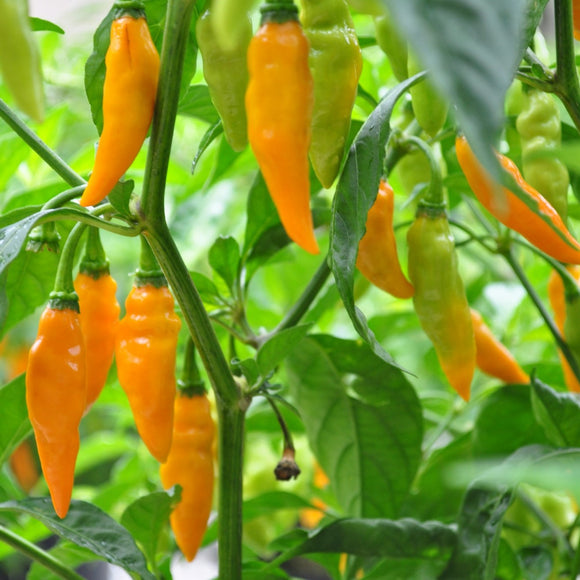This close-up image captures a pepper plant adorned with numerous peppers hanging from its green branches. The plant features dark green, teardrop-shaped leaves with prominent green veins. The peppers, varying in color from deep orange to green, hang from green stems attached to the branches. The majority of the peppers are a ripened deep orange, resembling Anaheim or serrano peppers in their slender and somewhat elongated shape. Towards the back and to the right of the image, many unripe green peppers, appearing more pruney, can be seen. One notable detail is a slightly brownish, rotted stem supporting one of the peppers. The background is filled solely with the lush green foliage of the plant.